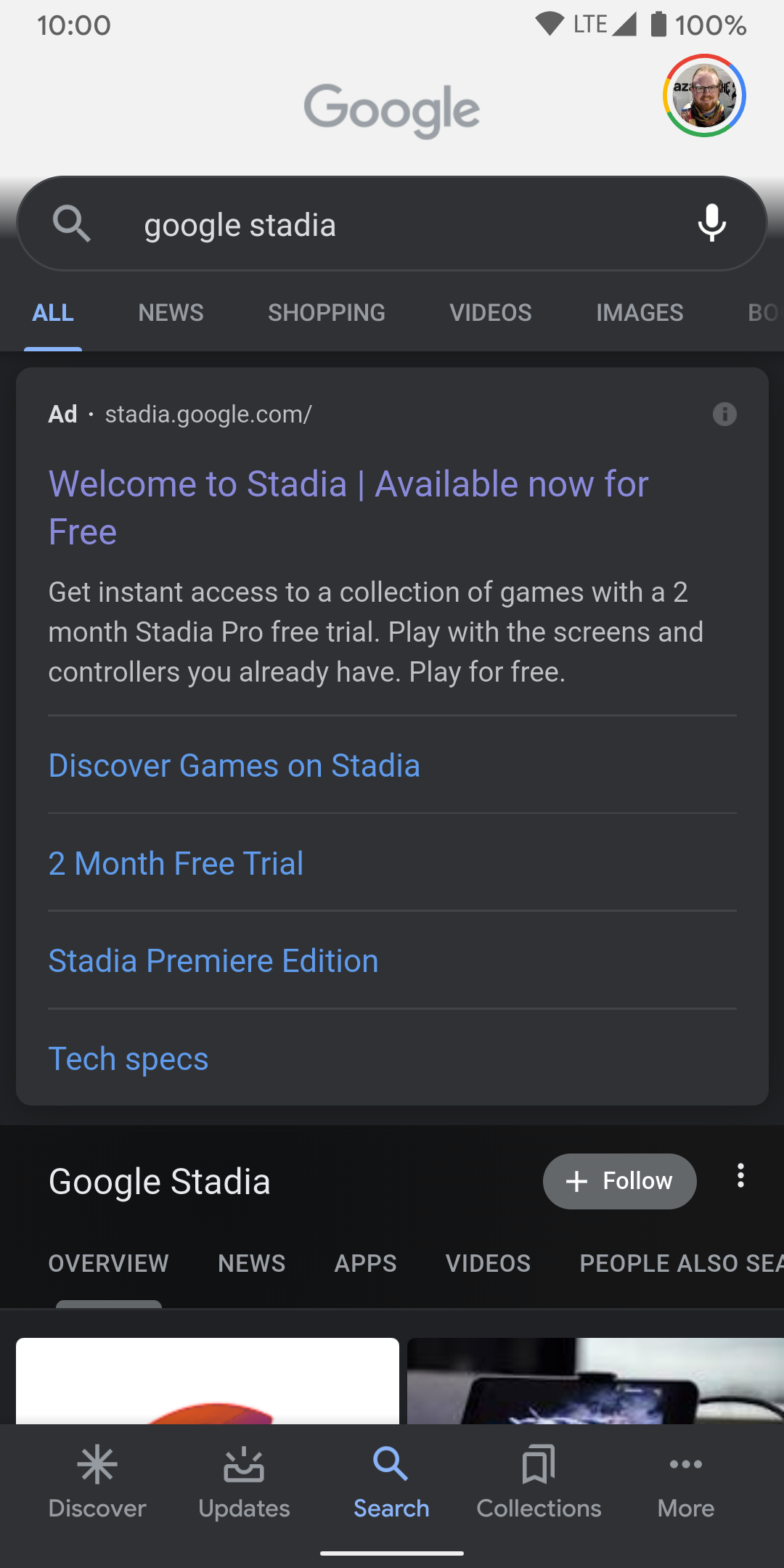This is a screenshot of a Google search page within the Google app, featuring a search for Google Stadia. At the top, the background is grey, with "Google" centered in grey text. On the far right, there is a circular profile photo, surrounded by the colors of Google's logo. 

Below, the search bar and the rest of the page have a black background. The first link is an advertisement in purple text, stating "Welcome to Stadia, available now for free," followed by a brief description of the product. Beneath this, there is a vertical list of Stadia-related options: 
1. "Discover Games on Stadia"
2. "Two Month Free Trial"
3. "Stadia Premier Edition"
4. "Tech Specs"

Further down, there is another listing for Google Stadia, with a "Follow" button on the right.